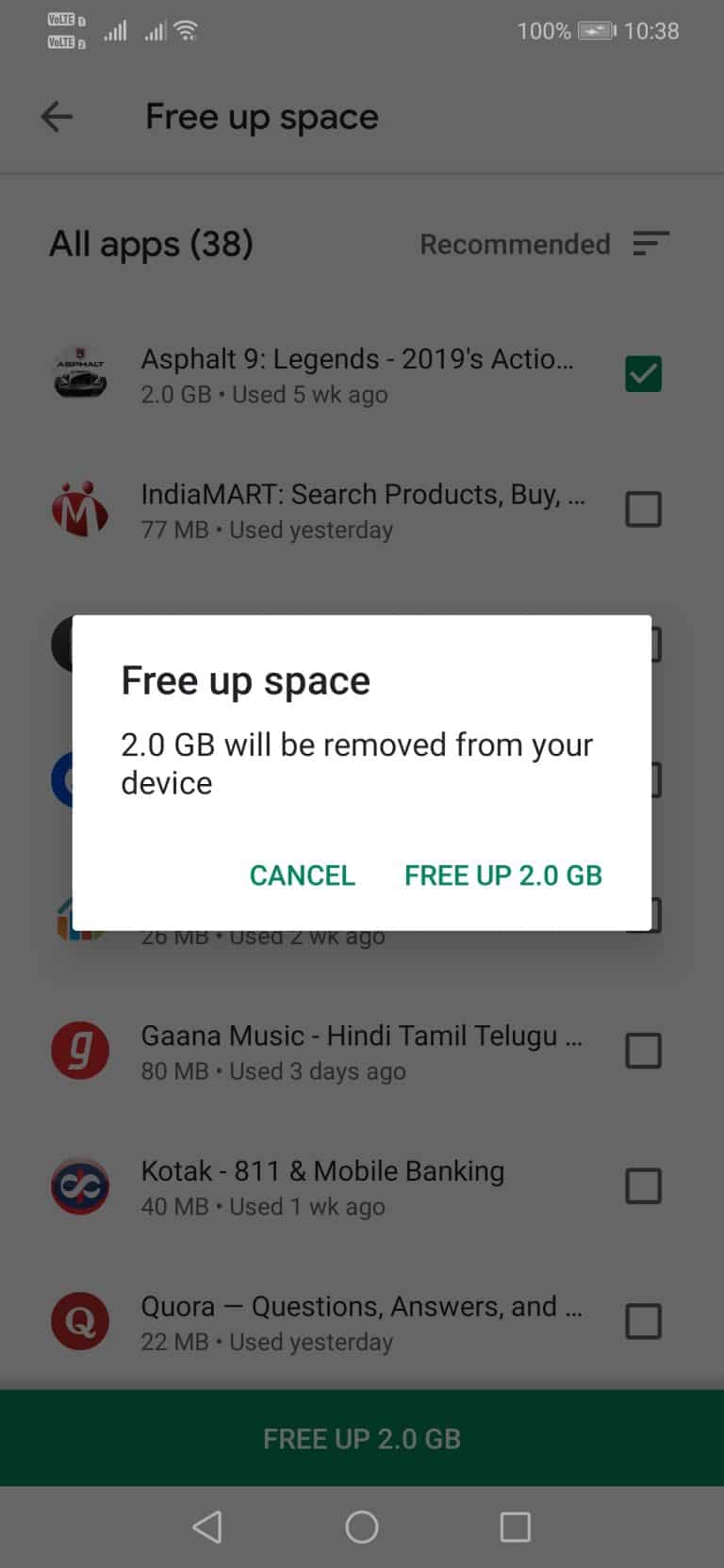This is a detailed screenshot of a smartphone displaying an app management page. The image includes a semi-transparent gray overlay with a white popup centered on the screen. The popup contains black text stating, "Free up space, 2.0 GB will be removed from your device,” along with two action buttons: "Cancel" and "Free up 2.0 GB." 

In the background, partially obscured by the overlay, various app details are visible. At the top of the screen, the status bar shows icons for battery (100% charged), Wi-Fi, and a timestamp of 10:38.

The app management page title, "Free up space," is displayed alongside a left-pointing arrow, followed by sections labeled “All apps (38)” and “Recommend.” Below are horizontal progress bars with diminishing lengths.

Further down, there is a list of apps starting with Asphalt 9: Legends, which occupies 2.0 GB and was last used five weeks ago. Next is IndiaMART, taking up 77 MB and used yesterday. Partially obscured by the popup are other apps such as Gaana (80 MB, used three days ago), KOTAK-811 (40 MB, used a week ago), and Quora (22 MB, used yesterday). 

Finally, the screen includes a green banner at the bottom that also says "Free up 2.0 GB," along with navigation icons for back (left-pointing arrow), home, and recent apps (square stop button).